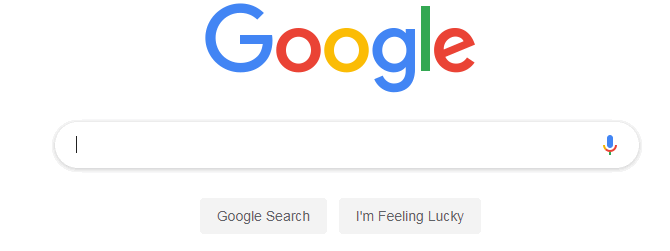A detailed and refined caption for the described screenshot would be:

"The image is a clean, uncluttered screenshot of the Google search page. Dominating the top center of the page is the iconic Google logo, with its colors arranged as follows: a blue 'G', a red 'o', a yellow 'o', a blue 'g', a green 'l', and a red 'e'. Directly below the logo is the prominent search bar, which contains a blinking cursor. Flanking the search bar are two icons: the 'G' shaped microphone on the right, indicative of voice search functionality. Beneath the search bar, centrally aligned, are two rectangular buttons. The left button reads 'Google Search' and the right button says 'I'm Feeling Lucky'; both inscriptions are in black text against a light gray background. The overall background of the page is a pristine white. No other elements, such as tabs or a browser address bar, are visible in this minimalist and instantly recognizable interface."